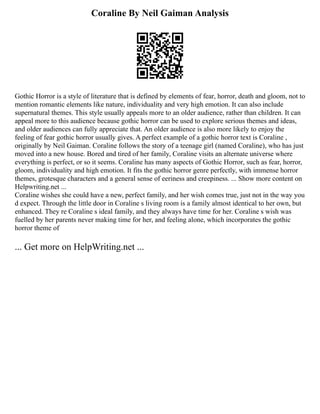The image is an information page with black text on a white background, centered around an analysis of "Coraline" by Neil Gaiman. At the top, it prominently features the text "Coraline by Neil Gaiman Analysis." Below this title is a QR code that can be scanned. Beneath the QR code, there is a block of smaller text, which begins with the line, "Gothic horror is a style of literature that is defined by elements of fear, horror, death, and romantic elements like nature or individuality." The text appears to delve into details about the book "Coraline" and its themes. At the bottom of the page, in larger text, it directs readers to "get more on helpwriting.net."